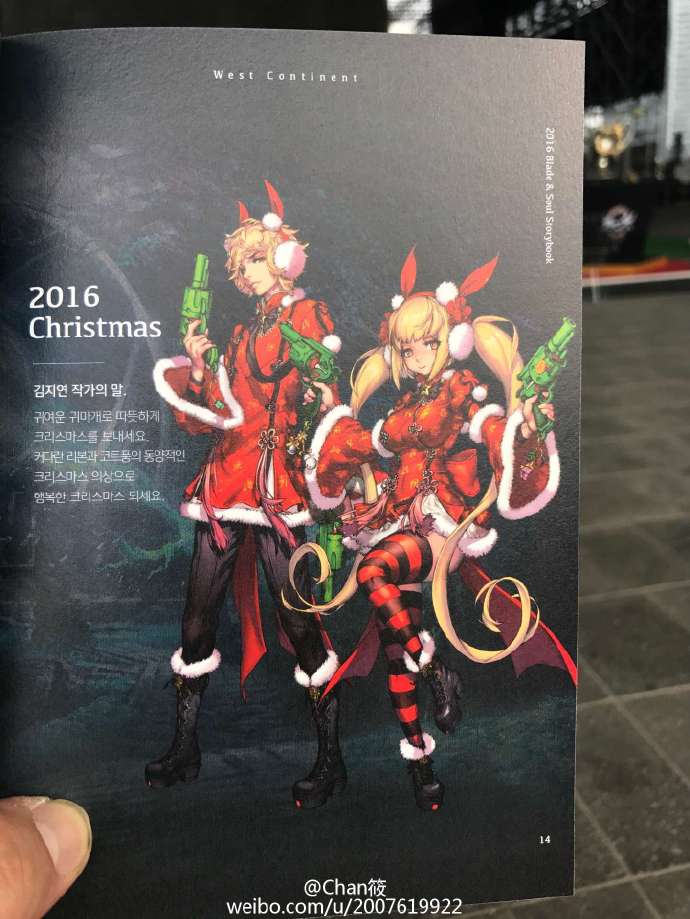In the vibrant winter scene, two female anime characters are dressed in festive Christmas attire. The character on the left is adorned in a red Christmas dress that seamlessly transitions into a skirt, complemented by white trim on the sleeves and hem. With a determined expression, she holds a green gun in her right hand, positioning it upright to showcase the right side of the weapon. Both characters sport adorable red Christmas-themed ear accessories, enhancing their holiday spirit. 

The character on the right wears a similar red Christmas dress, mirroring the festive design of her companion's outfit. She strikes a dynamic pose, gripping a gun in each hand - one in her left and the other in her right. Adding to her energetic stance, her left leg is bent upwards, causing her thigh to extend horizontally. The entire image exudes a blend of holiday cheer and action-packed excitement, brought to life by the detailed and intricate anime artistry.